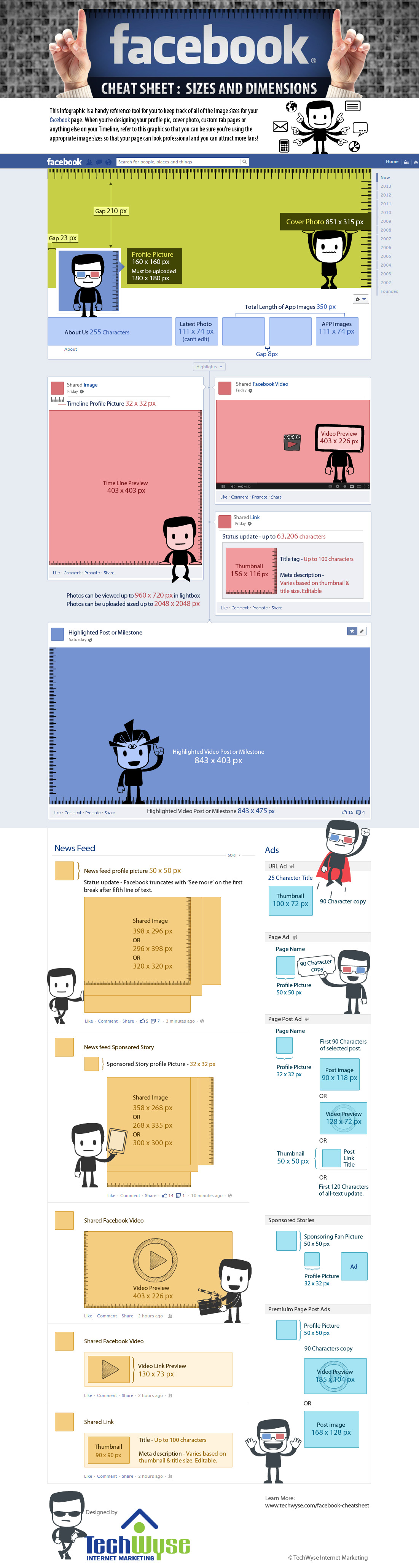The image, titled "Facebook Cheat Sheet: Sizes and Dimensions," is a detailed and comprehensive guide designed to help users optimize their use of Facebook's platform. Though the text is rendered in an exceptionally small font, making it unreadable, the diagram is visually intricate and filled with headlines, graphics, and various images. These elements illustrate how to effectively use and maximize space, leverage images, and utilize Facebook's features for optimal audience engagement.

The cheat sheet seems to cover a wide range of topics critical for creating a professional and impactful Facebook presence. It includes guidelines on background images, column headers, and specifications for posting images, videos, ads, and comments. The focus is on providing users with optimal dimensions and sizes to ensure that their content achieves maximum visibility and effect. This highly detailed guide is an invaluable resource for anyone looking to enhance their Facebook page's presentation and effectiveness.